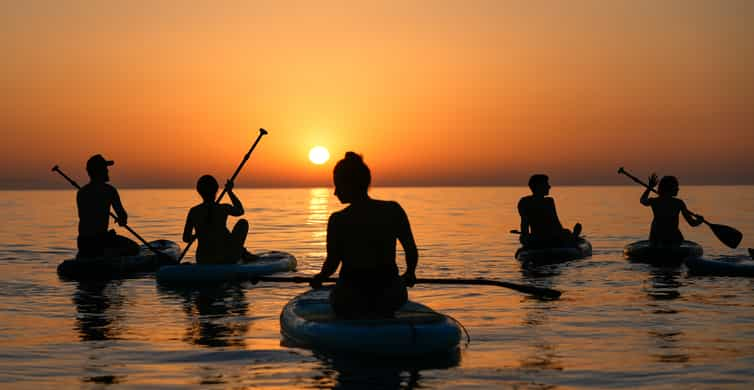At sunset, this beautifully composed photograph captures the enchanting scene of five young adults kayaking on a tranquil body of water, which could be a large lake or the ocean. The sky above transitions from a striking orange to a soft light yellow, with the sun depicted as a small dot nearing the horizon. The sun’s reflection casts an orange glow upon the rippled surface of the water, enhancing the serene atmosphere. 

In the foreground, the back silhouette of a woman with her hair in a bun is seen holding an oar on her lap. To her left, a man wearing a baseball cap is actively paddling besides another woman. To her right, another man rests his oar on his lap, while the woman beside him paddles with one hand raised. The silhouettes stand out against the vivid backdrop, encapsulating the tranquility and camaraderie of this moment shared in nature’s embrace.